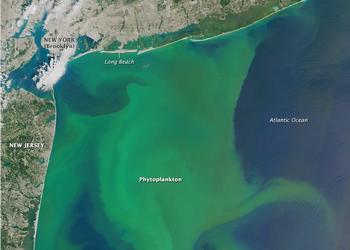This detailed satellite image showcases a large section of the Atlantic Ocean, primarily depicted in dark blue, with a striking green swirl in the water, suggesting the presence of algae or phytoplankton. The image labels the Atlantic Ocean prominently on the right side. Along the left and upper edges of the image, we can see the landmasses of New Jersey and New York, including specific areas such as Long Beach, New York City, and Brooklyn. The terrestrial regions are illustrated with various shades of brown and green, reflecting land features and vegetation. Notably, a river or waterway flows into the Atlantic Ocean from the bottom of New York, highlighting the connection between land and sea. Trees are visible along the edges of these waterways, adding detail to the landscape. The main focus remains the large, hurricane-shaped green area in the ocean, academically identified as phytoplankton, encircled by the surrounding land and oceanic expanse.